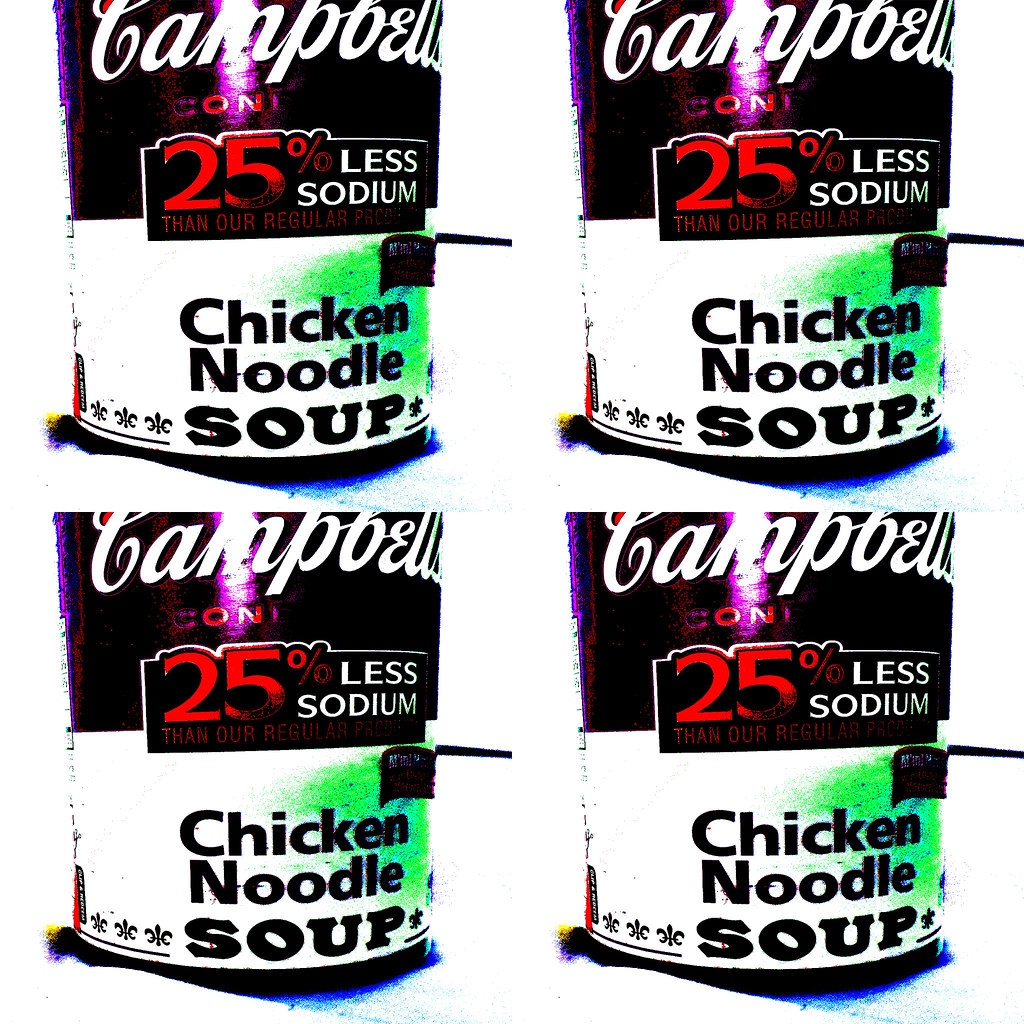This image showcases a stylized, Warhol-esque take on Campbell's chicken noodle soup cans. Four cans are arranged in two layers of two, with the upper cans partially cut off at the top, just above the word "Campbell’s." The cans exhibit a striking color inversion or filter: the usual red area is a purplish-black, and the bottom, which is traditionally white, retains its color but is overlaid with a greenish hue. The familiar yellow cloud to the right side is replaced with a light green version. The black lettering on the cans spells out "chicken noodle soup," accented by a red "C-O-N" for "condensed" and a prominent "25% less sodium" text block. The cans are slightly off-center, further emphasizing the unusual coloring and design elements, creating a visually captivating and repetitive motif.